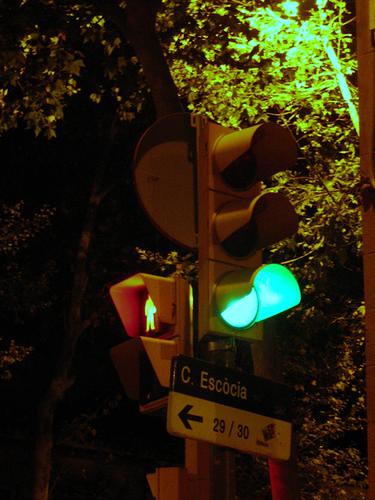In this nighttime photograph, a green-lit traffic light is seen slightly tilted to the right from a low angle. The traffic light features three arched sections, though only the bottom green light is illuminated. Below the traffic light is a horizontal black sign displaying "C. Escocia" and a white sign beneath it with an arrow pointing left and "29/30". To the left side of the traffic light, a pedestrian crossing signal shows a red "do not walk" indicator. The background features dark, illuminated foliage, suggesting additional lighting in the area. The sky is pitch black, enhancing the visibility of the illuminated signs and signals.